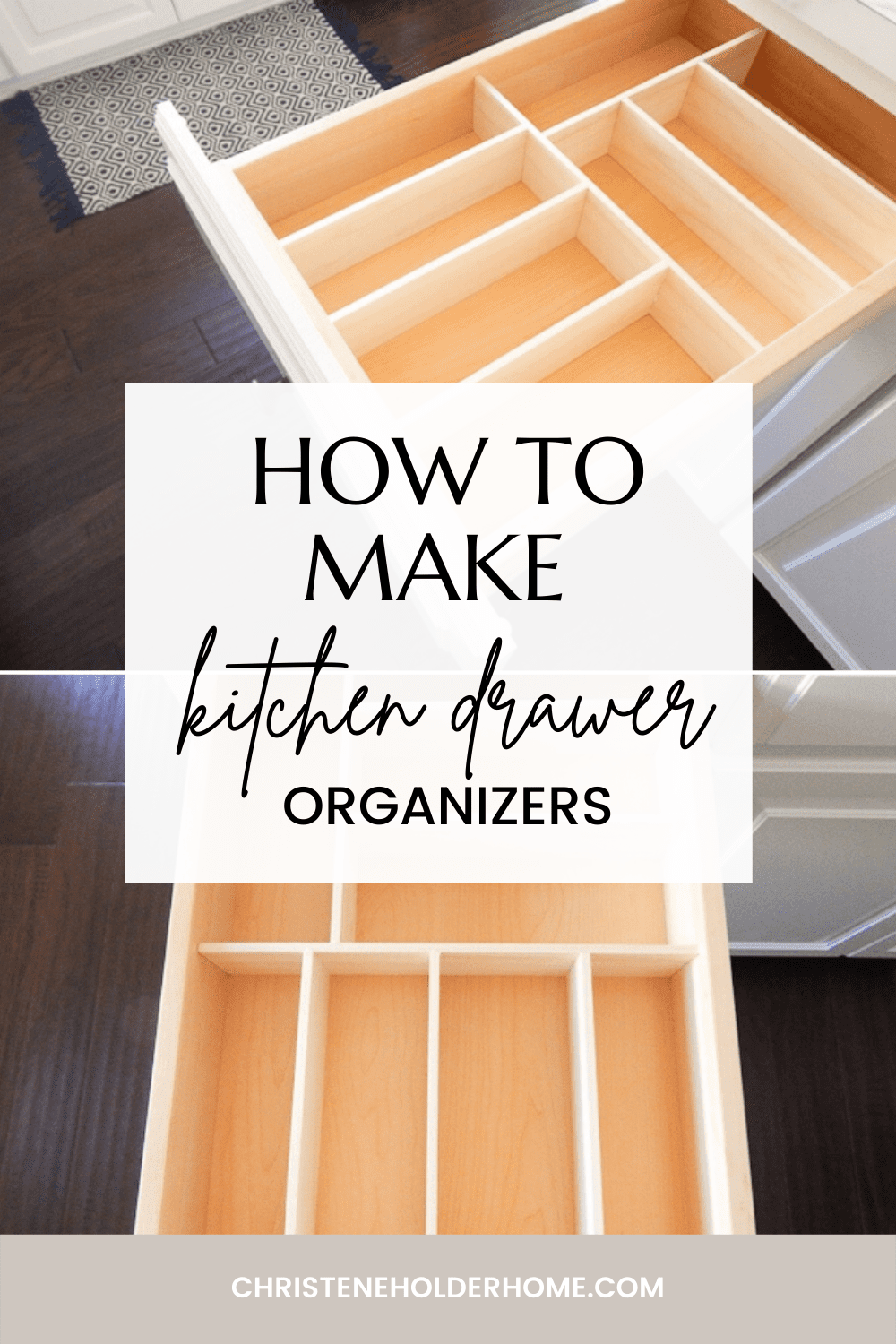The image, appearing to be a blog post or an advertorial from ChristineHolderHome.com, demonstrates the process of making kitchen drawer organizers. It features a central translucent whitish-gray box containing the text "How to Make Kitchen Drawer Organizers" in bold black font, with "Kitchen Drawer" in cursive. The background includes a montage of two photographs showcasing kitchen drawers with various organizational compartments. 

The top photograph provides a three-quarter view of a white kitchen cabinet with a single drawer pulled out, revealing dividers made of light-colored wood, likely used for utensils or silverware. This view also includes dark wooden flooring and a patterned rug with blue and white geometric designs and blue tassels. The bottom photograph offers a direct bird's-eye view of the same drawer, emphasizing the different configurations of the compartments. 

The overall aesthetic of the kitchen highlights white cabinetry, a dark wooden floor, and a black-and-white patterned mat. At the bottom of the image, a gray banner lists the website ChristineHolderHome.com in white capital letters, serving as a watermark. The images appear to be stock photos taken indoors, aimed at illustrating various ways to organize kitchen drawers efficiently.